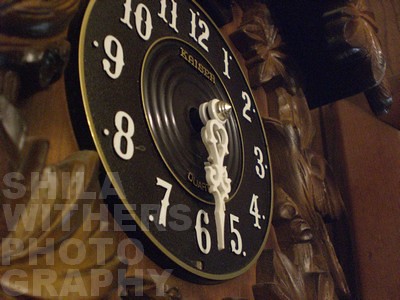This is a detailed photograph of a grandfather clock, predominantly showcasing its ornately carved wooden face. The wood, stained in a very dark brown, features intricate designs that resemble leaves and bells. The clock face itself is quite dark, framed by a gold trim around the outer edge and another gold circle towards the center. White numerals from 1 to 12 are clearly marked, with the white hour and minute hands set to 6:30. Just under the 12, the word "Kaiser" is inscribed in gold, while "quartz" appears above the 6, also in gold within the inner gold circle. A watermark in very bright white font is located in the bottom right of the photo, reading "Shilla Withers Photography." The background reveals a slightly off-brown wall.